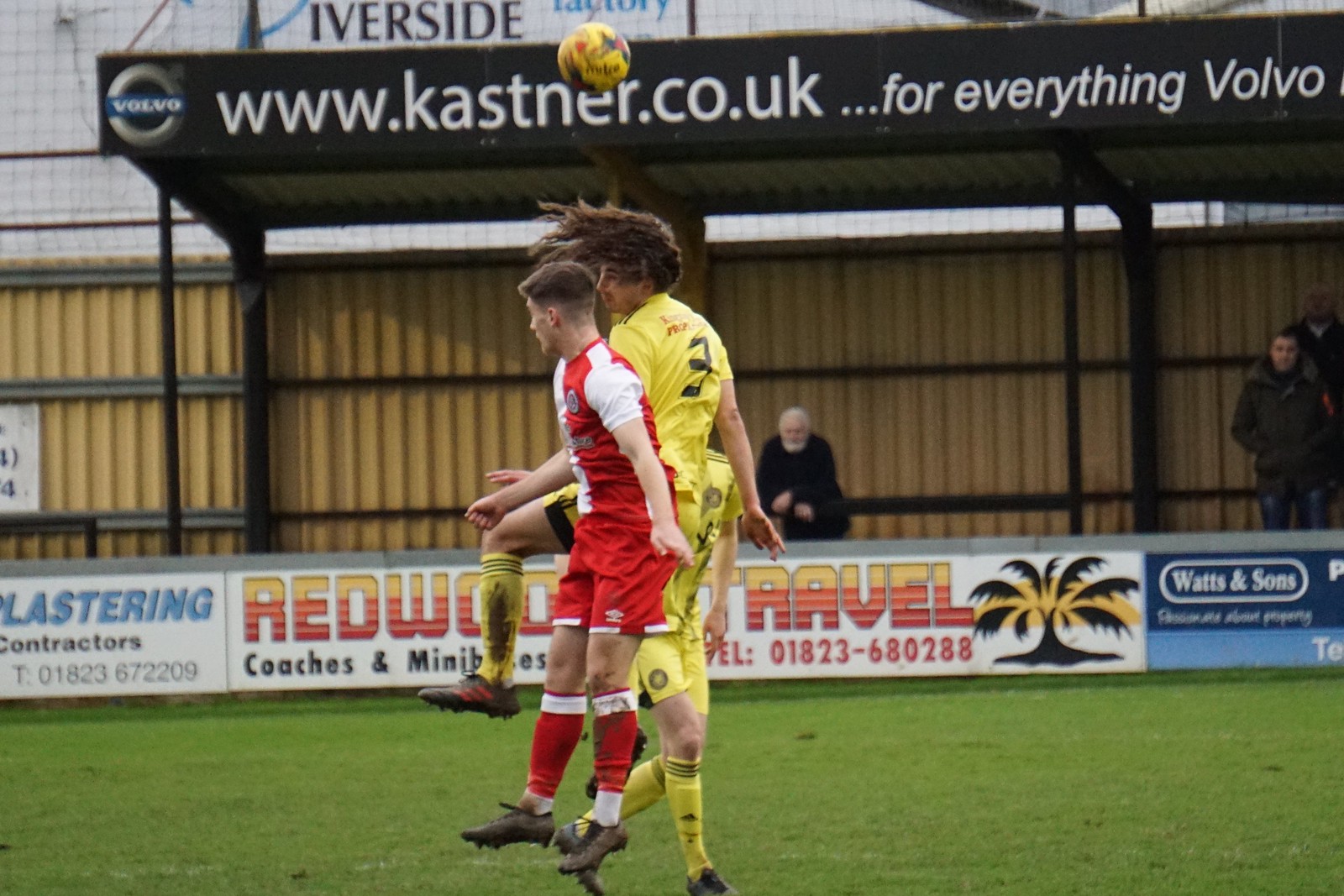In this dynamic action shot of a soccer game, possibly a practice session, the focus is on two players engaged in an intense moment on a lush green grass field. The player in the foreground, who is leaping majestically into the air to head the ball, is dressed in a red and white uniform, including a jersey, shorts with white trim, and matching socks, complemented by black cleats. His short brown hair and determined expression highlight his athleticism. To his immediate right, a taller player in a striking all-yellow uniform with black trim and numbers is also airborne, reaching even higher as he attempts to challenge for the ball. The yellow-clad player has long brown hair flowing behind him, emphasizing the motion of the jump.

In the background, another yellow-uniformed player stands on the ground observing the duel, creating a layered depth to the image. The scene is set against a backdrop of various advertisements. A brown fencing wall runs horizontally, adorned with signs such as "Plastering Contractors," "Redwood Travel – Coaches and Minibuses, Telephone 01823-68-0288," and "Watson Sons."

Further behind, under a corrugated metal overhang supported by metal bars, two men stand and watch the game. Above them is an advertisement that reads "www.castner.co.uk for everything Volvo," accompanied by a prominent silver and blue Volvo logo. The overall composition not only captures the action and intensity of the soccer match but also the commercial and human elements present at the venue.